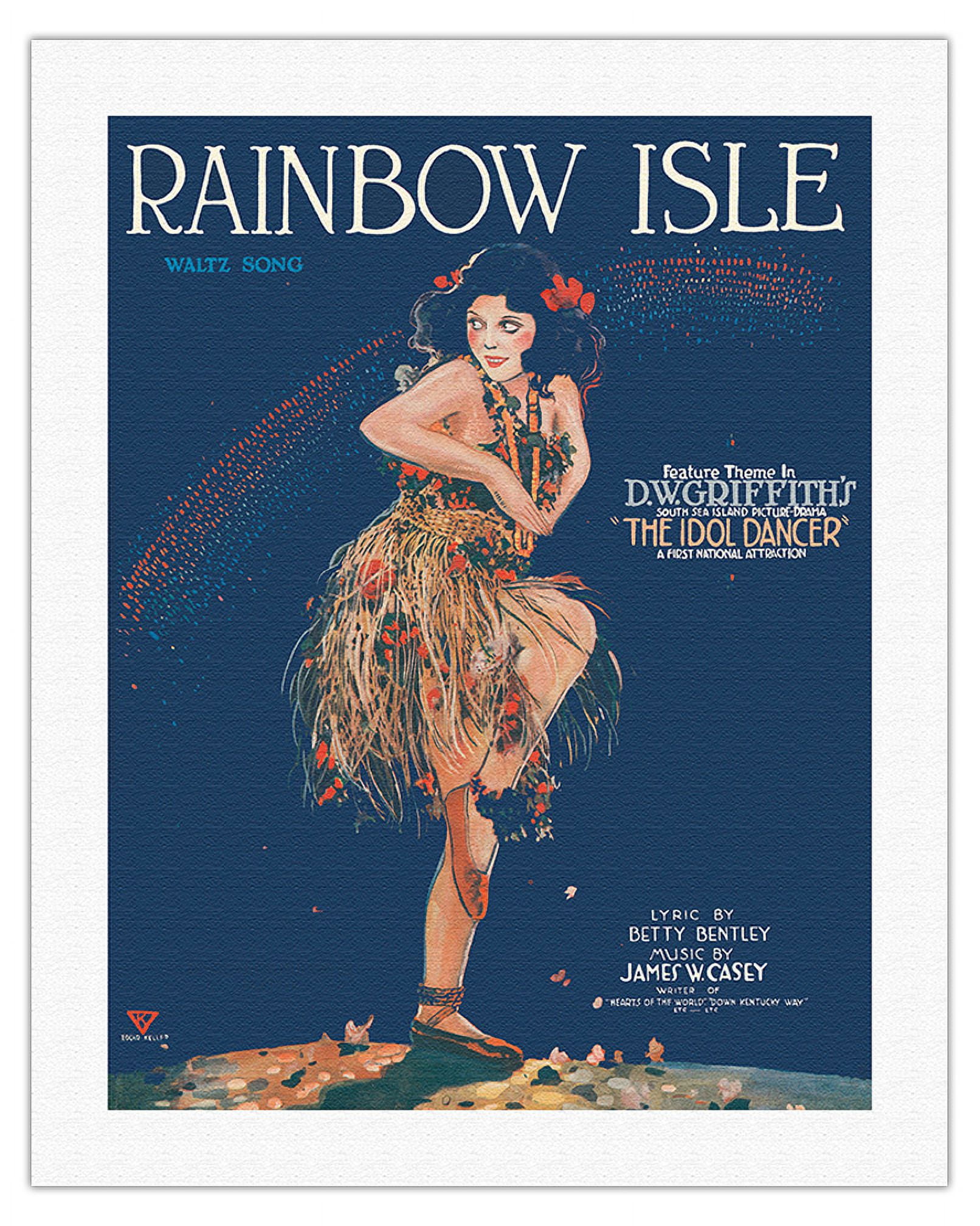The image is a vintage artistic promotion poster, possibly for sheet music, titled "Rainbow Isle" at the top in prominent text. Just below the title, in a smaller blue font, it says "Walt Sasson." Dominating the center of the illustration is a woman dressed in traditional Hawaiian attire, featuring a stringy grass skirt adorned with red flowers. She also has red flowers adorning her shoulder-length, poofy black hair. The woman, depicted as dancing, has blushed cheeks, red ballet slippers tied around her ankles, with her left leg bent at the knee and her other leg flat on the ground. Her right arm is raised at a right angle across her chest, and her gaze is directed towards the left. The background of the illustration is navy blue. To the right of the woman, text reads "Feature theme in D.W. Griffith's South Sea Island Featurama 'The Idol Dancer,' a first national attraction." In the bottom right corner, additional text states "Lyric by Betty Bentley, Music by James W. Casey," with more illegible text below that due to its small size.